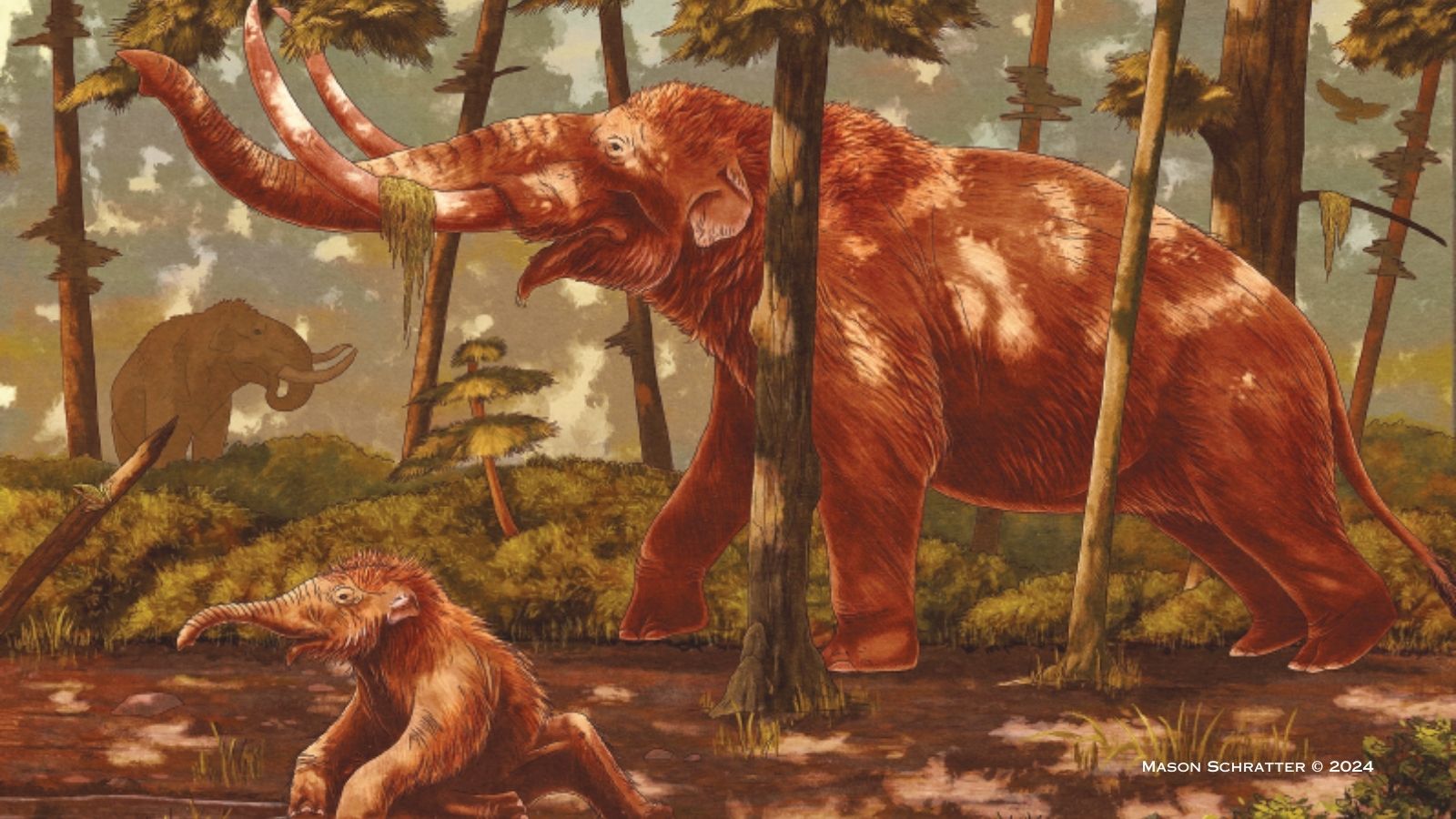The image is an artistic illustration by Mason Schrader, dated 2024, depicting an ancient, prehistoric scene nestled within a dense forest. In the foreground stands a large brown mammoth with long, curved tusks and a shaggy coat, extending its trunk upwards to graze on the leaves of thin-trunked trees. Next to it, a baby mammoth is sitting on the brown dirt, likely its offspring. In the distant background, another mammoth is visible, standing among the verdant foliage with its large tusks prominently displayed. The scene is rich with greenery; tall trees with leafy canopies surround the animals, creating a lush, forested setting. The sky above is a deep, bluish-green hue, adding to the ancient and serene atmosphere of the illustration. The artist’s name and the year “Mason Schrader, 2024” are clearly marked in the bottom right corner.